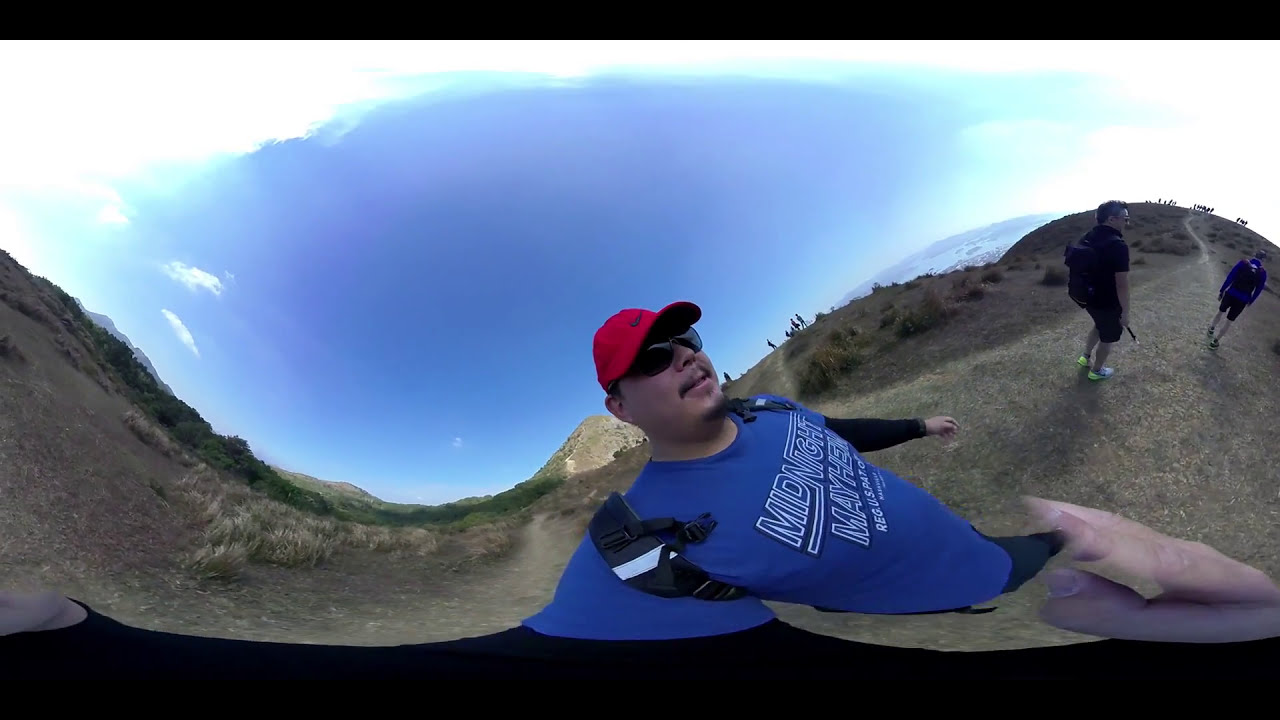This image depicts a man standing outdoors on a hilltop trail beneath a vivid blue sky surrounded by a bright white light. The man, possibly of Asian or Hispanic descent, is wearing a red baseball cap, dark sunglasses, a tiny mustache, and a blue t-shirt with white-outlined lettering. He also has black straps crossing from his shoulder to his armpit and appears to be holding the camera with his left hand above his left shoulder, creating a selfie at an unusual angle. The photograph is notably warped, with three distinct bubble-like distortions across the image.

In the background, the trail meanders up a hill, where two additional people are visible, albeit small and somewhat indistinguishable due to distance and perspective. One person, possibly carrying a backpack, is dressed in shorts and a t-shirt. Another smaller figure, whose age or size and attire are unclear, is present at the very right edge of the photo. The landscape features two dramatic hills flanking the scene, with one hill descending into the center on the left side and another hill rising on the right. These hills frame the dirt pathway which the group is traversing.